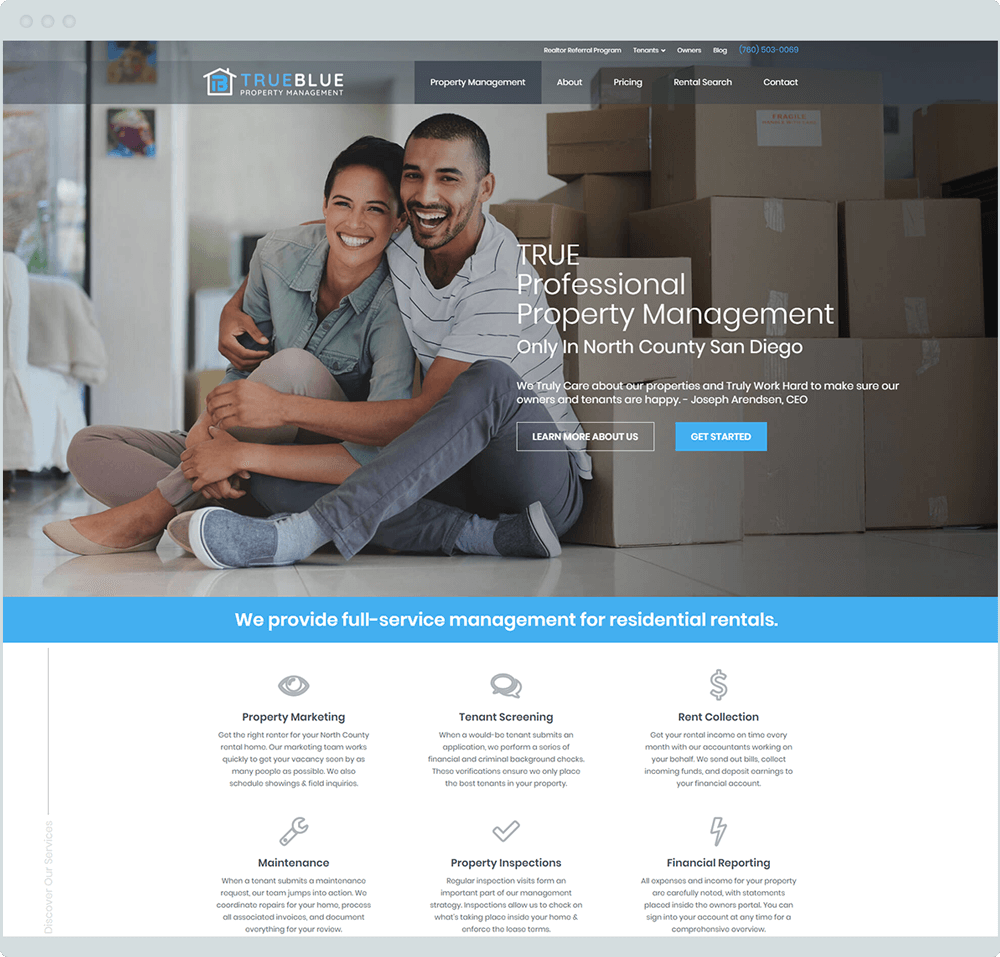This cropped image showcases a mock-up design of a website, identified by the presence of a browser bar at the top featuring three dots on the left and a gray bar, devoid of any other icons. Below this bar is the logo and title "True Blue Property Management," where "True" is in blue and "Blue" is in white. The logo features a white house graphic with the initials "T.B." inside. 

To the right are five clickable menu options in white text. Dominating the page is a large splash image, prominently displaying the text "True Professional Property Management, only in North County, San Diego." The image itself shows two people sitting on a clean, tile-floored surface with white walls, leaning against a large stack of moving boxes, suggesting a recent move-in.

Beneath the image is a blue banner with white text that reads, "We provide full-service management for residential rentals." Below this banner is a grid layout, organized into two rows of three icons each, representing different aspects of the property management services offered. These icons include a cash icon, a wrench icon, and a lightning bolt icon, among others, and are accompanied by center-justified paragraphs that explain each service in detail.